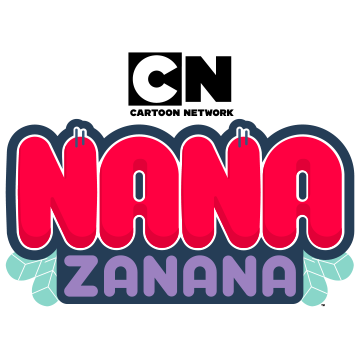The image showcases a promotional ad, possibly for a Cartoon Network show, against a plain white background. At the top center-left, there is a distinctive black square featuring a large white "C." To its right, a thick black "N" completes the Cartoon Network logo. Directly beneath, in smaller black text, it reads "Cartoon Network." Below this, in large red bubble letters with a thin white outline and a thicker dark blue border, the word "NANA" stands out prominently. Notably, the second humps of both "N"s feature two vertical gray stripes. Emerging from the bottom corners of "NANA" are mint green leaves, adding a playful touch. Underneath "NANA," set against a dark blue background, bold purple text spells out "ZANANA."